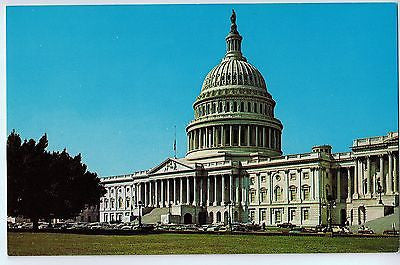This horizontally aligned, rectangular photograph appears to be a vintage shot of the U.S. Capitol building, likely dating from the 1970s given the quality and saturation of the colors. The Capitol stands prominently against a clear, vivid blue sky that occupies the entire upper half of the image. The structure is characterized by its large stone columns and an iconic domed top with a pointed tip. Its stone facade appears to be a grayish-brown or beige-off-white color. An expansive, manicured green lawn stretches across the bottom foreground of the picture. On the right side of the lawn, the grass is bright green, fading to a brownish hue on the left. Numerous cars are parked in front of the building, hinting at a time when security was less stringent. A dark silhouette of a large tree is discernible on the left side, adding contrast to the scene. The overall atmosphere is tranquil, with no visible people except for a few indistinct figures that might be present on the far right side.